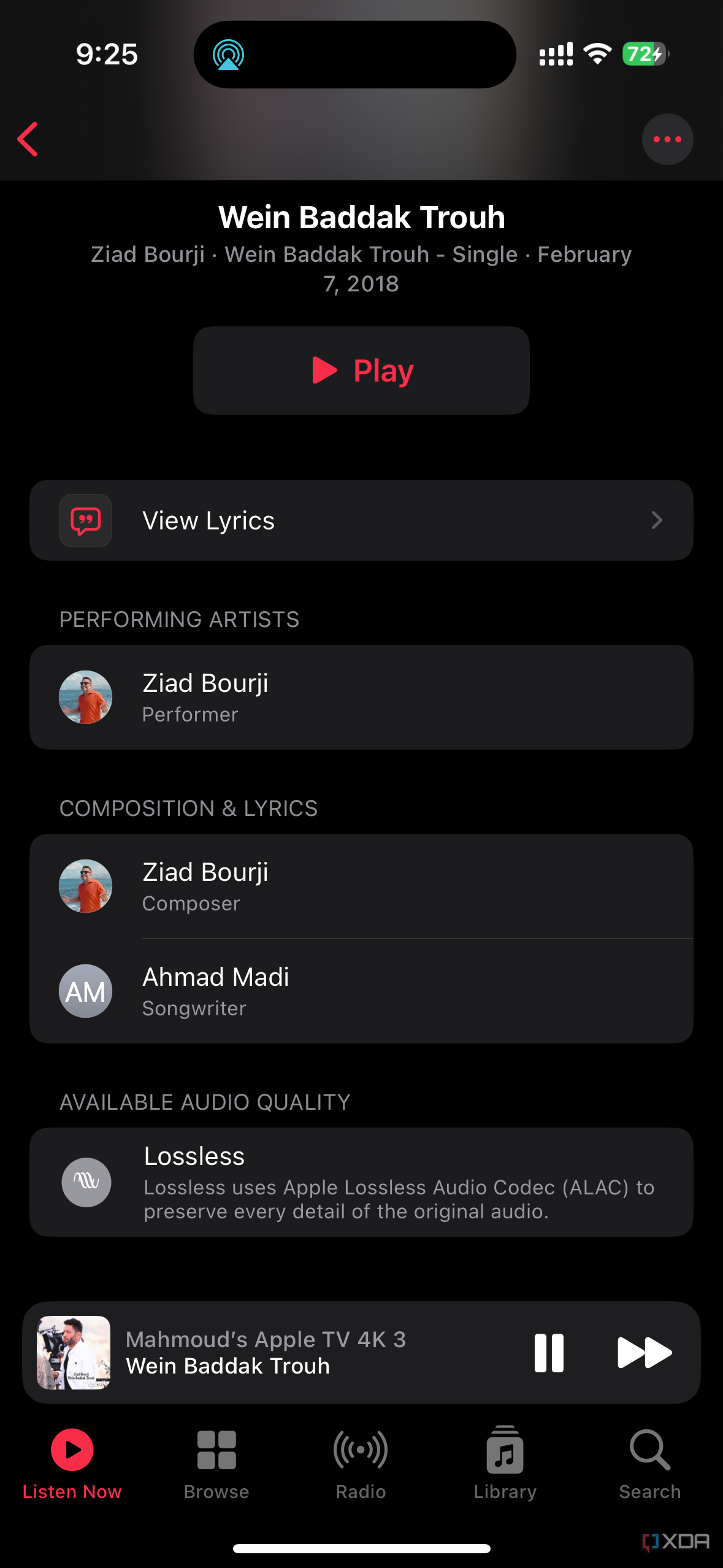At the top left, the image prominently displays the time "9:25" in small, bold, white lettering centered within the area. Adjacent to this, there's a large black oval shape situated slightly to the left, accompanied by an aqua triangle positioned to its left. Extending from this triangle are several lined circles. Moving towards the right of the image, there are four horizontal bars, segmented by a black line running across the bottom. Just beside these bars is a Wi-Fi symbol, and next to it, a battery icon showing a 72% charge.

The background features a gradient, starting with light gray in the center and transitioning to black towards the edges. Positioned towards the left, a red arrowhead points leftwards. On the right side, there's a light gray circle containing three red dots in its center.

Dominating the middle portion of the image is a section with a black background and bold, white text that reads "WEIN BADDADAK TROUH." Below this, in smaller, light gray font, it says "ZIAD BOURJI," followed by a bullet point, then the text "WEIN BADDADAK TROUH - single," another bullet point, and "February 7, 2018."

Towards the bottom, there's a dark gray button with rounded rectangular edges, featuring a play icon that straddles between a dark pink and red color. Below this, the option to 'View Lyrics' is visible, and to the left of this option is a comment or message icon, matching the reddish hue of the play button.